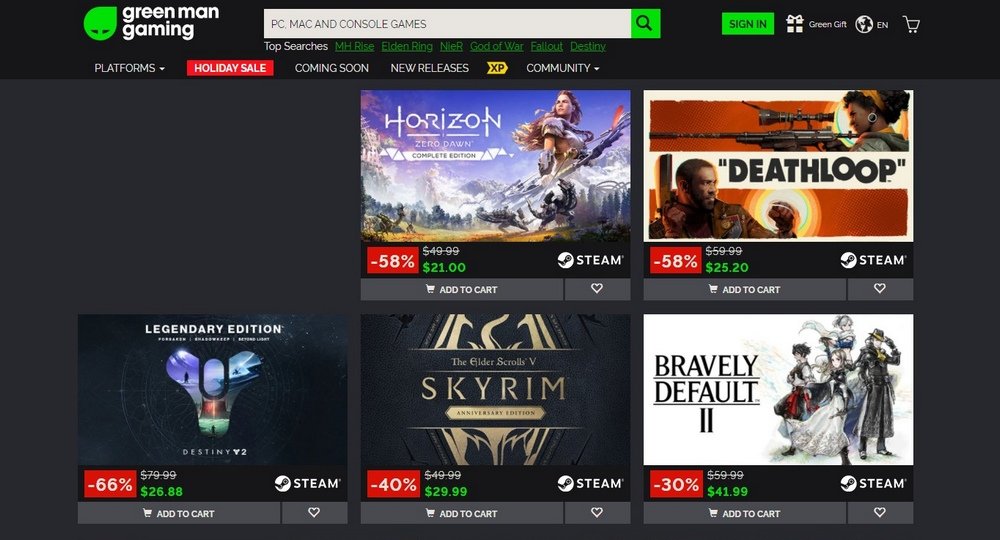The image depicts a webpage from a digital game store. At the top center is an illustrated green icon resembling a circle with a small point, featuring two eyes that give it a character-like appearance. The search bar, prominently highlighted in green, lies beneath this icon. Above the search bar, there is a green "Sign In" button. Below it, various navigation categories are listed, including Platforms, Holiday Sale, Coming Soon, and New Releases.

Adjacent to these categories is an XP and a yellow image symbol, followed by a "Community" section featuring a drop-down menu. 

The lower part of the image showcases several game cover art thumbnails. The first thumbnail slot is blank, suggesting an image might be missing. The second thumbnail is for the game "Horizon," depicting a woman standing atop a snowy landscape while holding a sword. 

The next thumbnail displays "Deathloop," featuring characters armed with guns. The fourth game is identified as "Legendary Edition" and shows an abstract graphic resembling two circles at the bottom and two forming a head-like shape at the top. Adjacent to this is the iconic "Skyrim" logo, presented with gold text on a black background. 

The final thumbnail is for "Bravely Default II," although specific visual details for this cover are not provided.